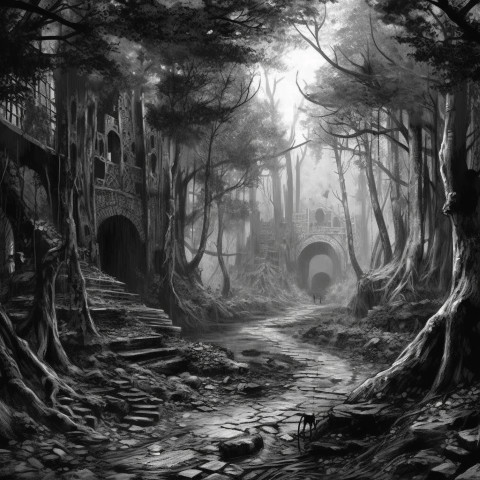The black and white digital image depicts an eerie, abandoned city nestled within a dense forest. Dominated by dark tones due to the abundant overgrown and leafless trees, the scene evokes a gothic sense of mystery. In the center, a winding stone pathway serves as the focal point, guiding the viewer's eye through the composition. To the left, a multi-leveled stone building reminiscent of a castle features numerous artistic doorways and staircases, along with a mix of small and large windows. The entire structure appears in ruins, yet holds an air of grandeur. The trees in the foreground have large, intrusive root systems that almost blend into the stone path, adding to the untamed atmosphere. In the background, partially obscured by shadow, an arched stone bridge or possibly an entryway stands out, constructed from a blend of cut and natural stone. The diffuse light filtering through the trees in the background casts an ethereal glow, subtly illuminating the scene and enhancing its haunting beauty.